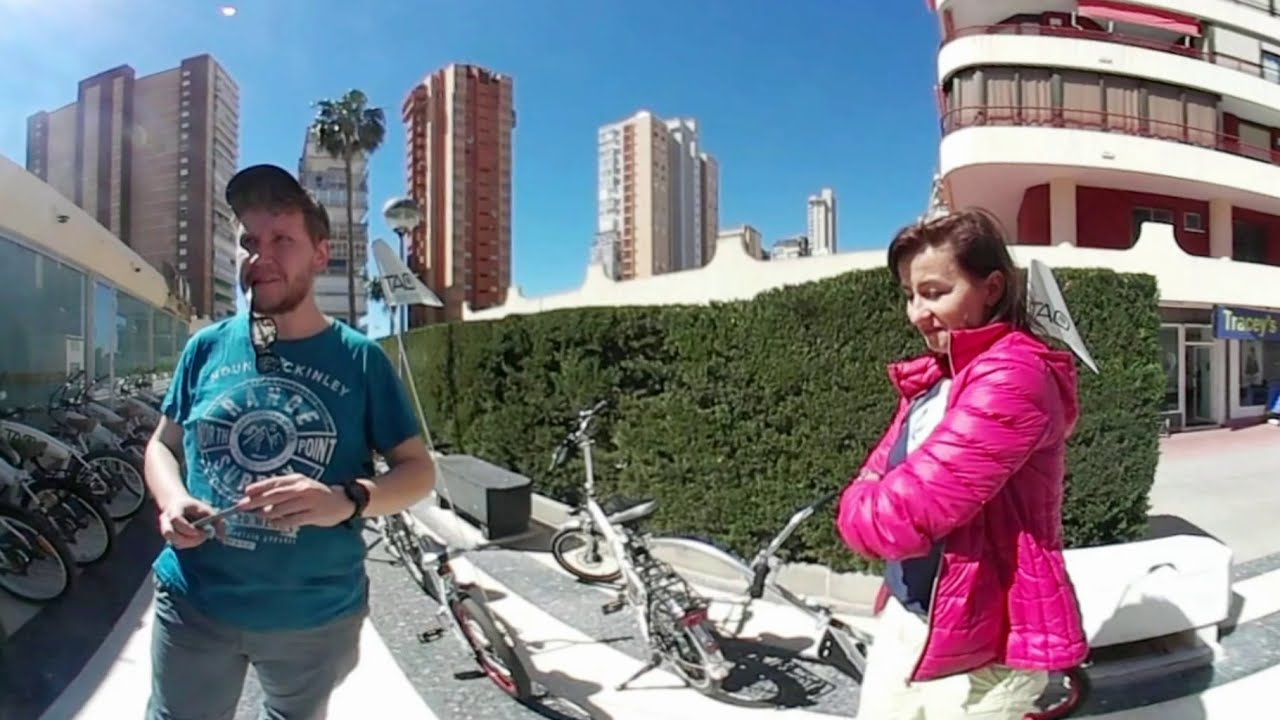In this vibrant, sunny, outdoor scene, we see two individuals standing in the foreground. The gentleman on the left is wearing a turquoise short-sleeved shirt adorned with various graphics and writing. He has a hat on his head, a beard, and has sunglasses dangling from his mouth while holding something with both hands in front of his waist. He pairs the shirt with grey pants. To his right, there is a line of bicycles, some standing upright and others lying on the ground, with tall hedges behind them. A stone bench can be seen to the right of the gentleman.

Adjacent to him on the right stands a woman with light skin and dark short hair. She is dressed in a puffy, purple-pink jacket over a white t-shirt, with her arms crossed and her gaze directed downward. In the background, tall, thin skyscrapers, likely around 40 stories high, rise into a clear, dark blue sky, lending an urban backdrop to the suburban setting. The high-rise buildings vary in color from tan to grey shades. The overall atmosphere is bright and lively, with emphasis on the contrasting colors and textures present in the scene.